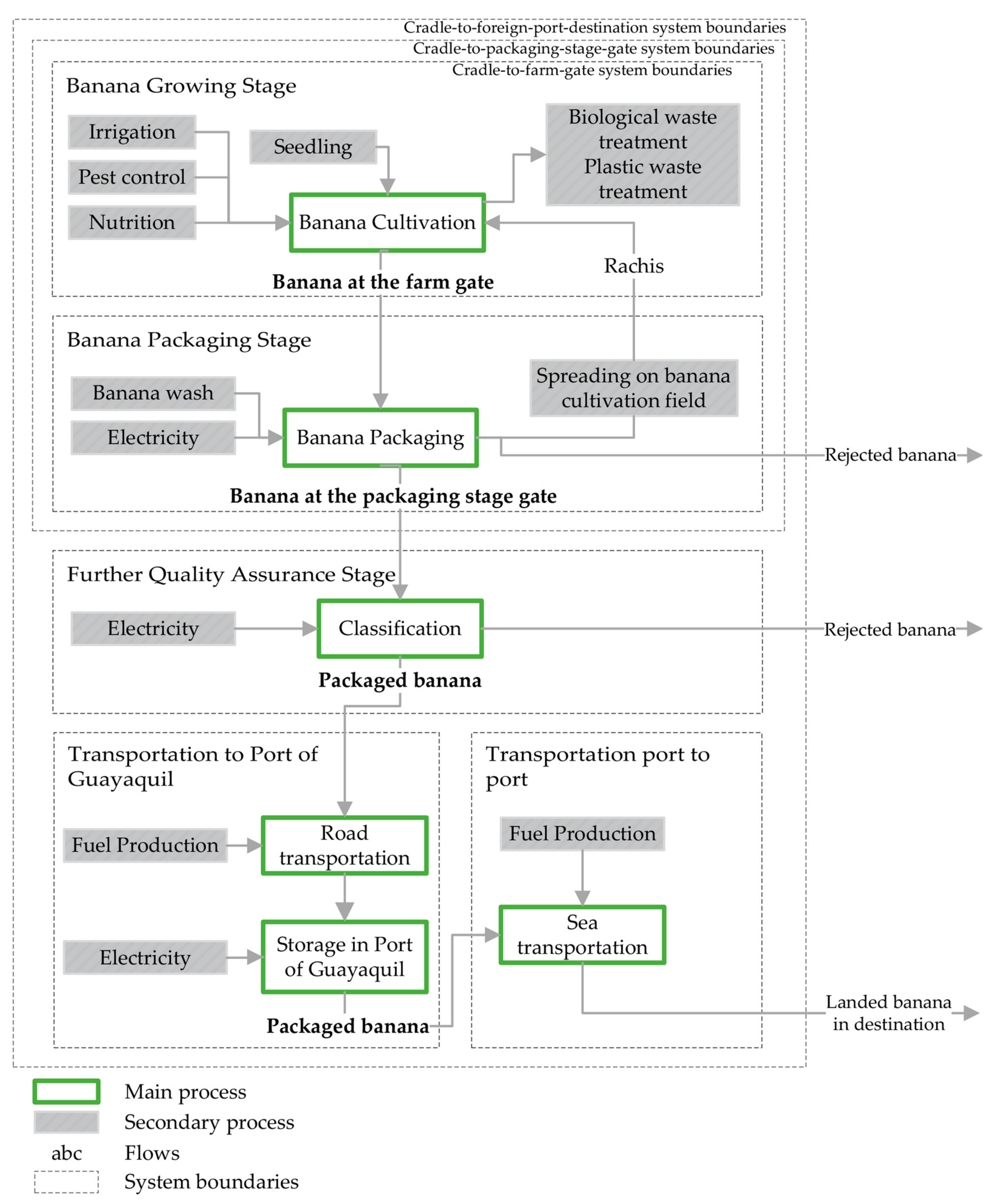The image is a detailed text infographic illustrating the stages of banana cultivation, packaging, classification, and transportation in a portrait orientation. The infographic is outlined by a broken black line, with several broken black segments inside, creating a structured flowchart. 

At the top, in black letters on a white background, the "banana growing stage" is highlighted; it includes components like irrigation, pest control, nutrition, and seedling, all in gray rectangles. This section flows into a green-bordered white area labeled "banana cultivation," which is connected to processes such as biological waste treatment and plastic waste treatment.

Below this, the "banana at the farm gate" stage appears, detailing banana washing and packaging activities. The flow continues to the "banana packaging stage gate," moving through further quality assurance steps, electricity usage, and classification processes, which are also encompassed by green borders. 

After classification, packed bananas proceed to "transportation to port of Guayaquil," incorporating road transportation fueled by fuel production. Subsequent stages include electricity utilization, storage at the port, and eventual "sea transportation." The journey concludes with bananas reaching their "landed banana destination."

The infographic also meticulously indicates rejected bananas at different stages, ensuring comprehensive process tracking. A legend key at the bottom left explains the symbols: green lines denote the main process, gray lines signify secondary processes, and dotted white areas outline system boundaries. 

This structured flowchart effectively delineates the entire journey of bananas from growth to their final shipment destination.